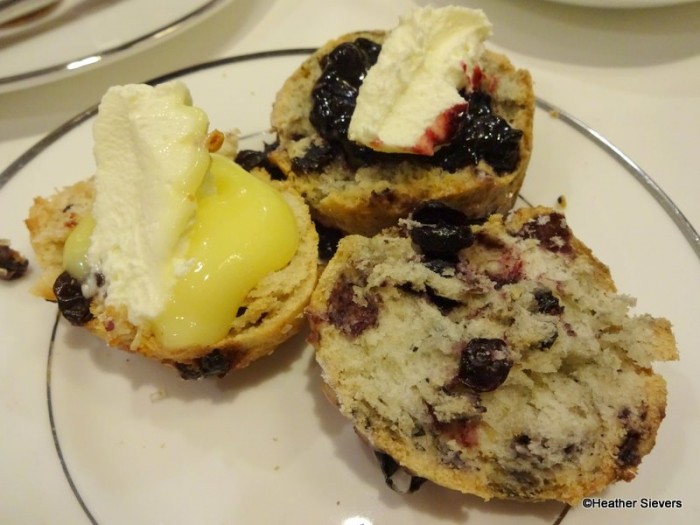The image depicts a close-up, horizontal rectangular photograph of a round porcelain plate with an ornate silver rim and an additional inner silver circle. The plate, centrally positioned yet slightly towards the bottom of the frame, holds three halved circular pastries that resemble blueberry scones. These pastries, with golden-brown crusts and flaky, white insides, are marked with vibrant purple stains from blueberry filling. The half in the forefront is plain, showcasing its simple form, while the others, positioned slightly behind and to the right, are adorned with various toppings. One of the halves has a generous amount of brie and a cluster of blueberries, whereas another is topped with a yellow viscous liquid, possibly jam, and a solid white substance that looks like butter. The overall setting appears to be in a kitchen or restaurant, with hints of other plates in the background. The colors in the image include shades of white, gold, purple, red, and yellow, creating a rich, appetizing visual. The name "Heather Sievers" is visible in text at the bottom right of the image.